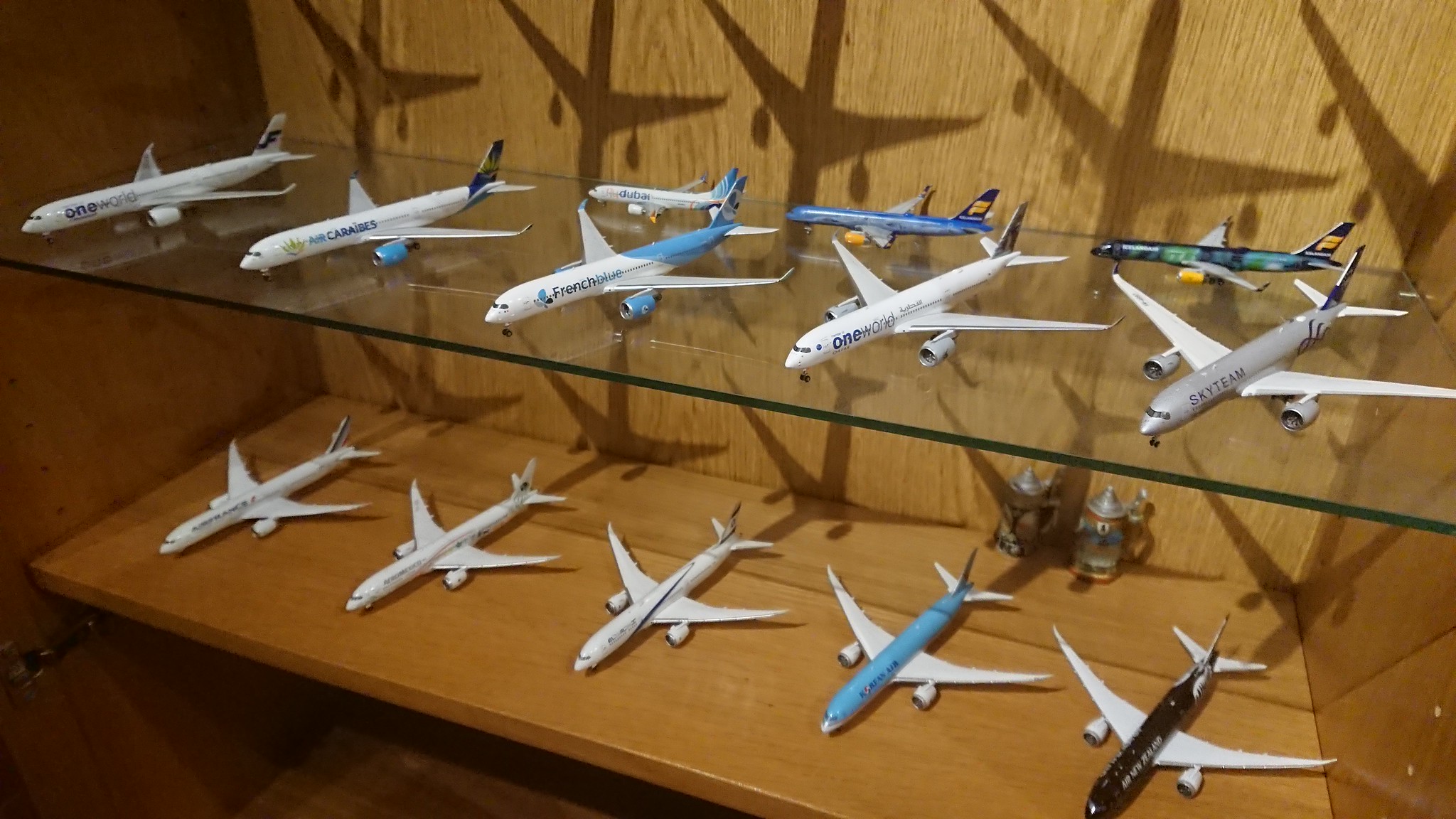The image showcases a meticulously arranged collection of approximately 12 to 13 model airplanes displayed within a cabinet that features two distinct shelves. The bottom shelf, made from wood, holds a row of five predominantly white planes, with notable exceptions such as a blue plane with white wings and a black plane with white wings. Two cans are visible towards the right edge of this wooden shelf, adding an extra layer of detail to the setting. The top shelf is crafted from glass and hosts five planes in the front row, mostly in white, with a gray one standing out among them. Behind these front planes, three smaller models are positioned sideways, each displaying unique color patterns: the middle one is blue, and the side planes exhibit a combination of blue, yellow, green, and black with distinct design elements on their wings and tails. Additionally, some of the planes are branded with logos and names such as Sky Team, One World, and French Blue, giving a commercial aviation touch to the collection. This well-organized display, captured from a right angle through a wide-angle lens, highlights the intricate detailing and varied designs of the miniature aircraft.